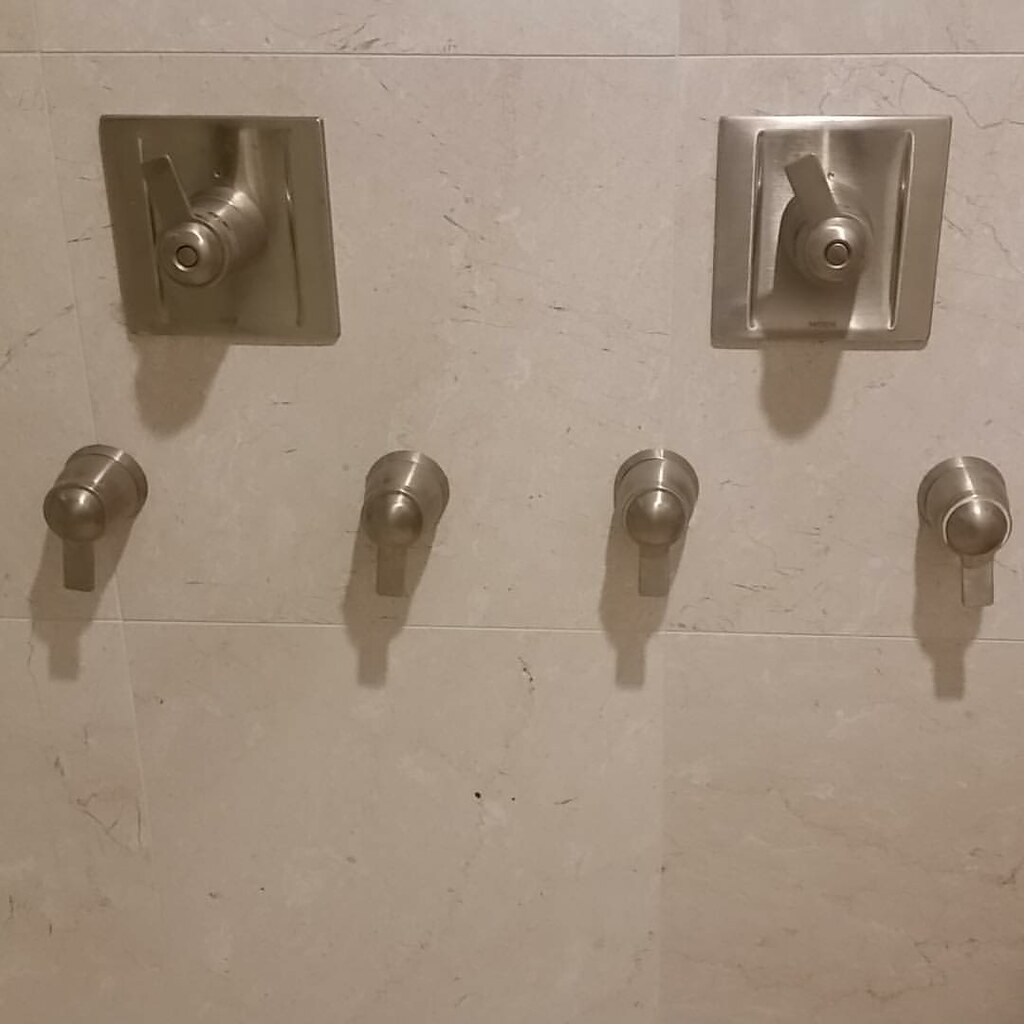This image captures a large, white, tile wall that appears to be from a communal shower area, possibly in a gymnasium, dormitory, or military facility due to its utilitarian design. The level of detail in the image allows one to discern a textured, travertine-like finish on the tiles. Near the top of the wall, there are two parallel, rectangular, silver panels, each inset with a central lever that resembles a shower control handle used for regulating water temperature by moving left to right. Below each panel, there are four evenly spaced, silver knobs, smaller than the levers above, aligned in a horizontal row. These knobs, which resemble doorknobs, reflect off the tile wall, adding to the metallic gleam of the installation. Although none of the fixtures are labeled, one might infer that the levers control water flow or pressure, while the lower knobs adjust the temperature. The orderly arrangement and repetition of the fixtures contribute to the impression of a shared shower facility.